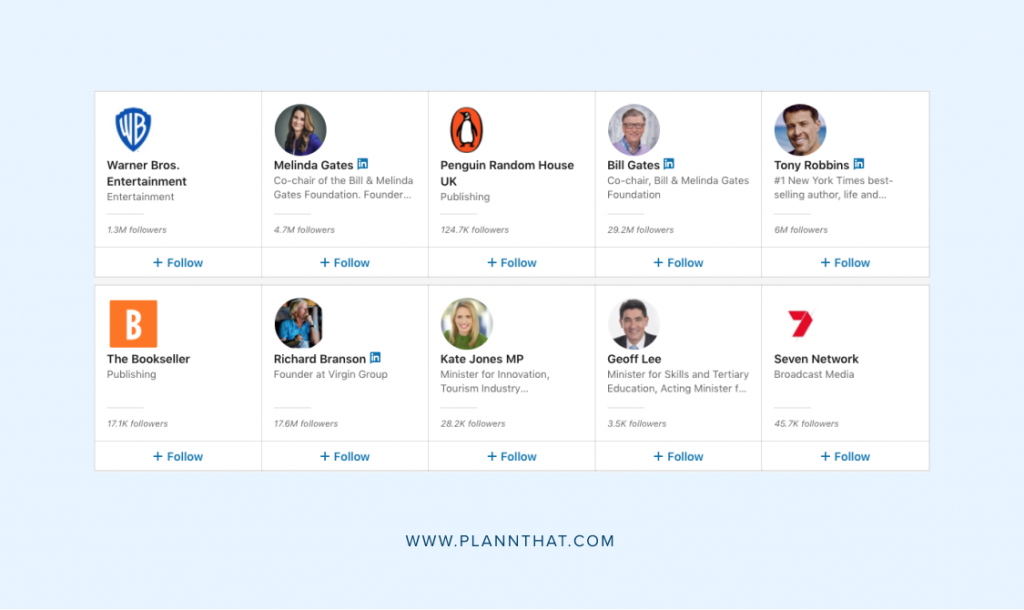This image, sourced from www.plannthat.com, features a light blue box containing two rows of clickable squares. Each of these ten squares includes a distinct icon, a title, follower count, and a "Follow" button. 

In the top row, the featured profiles are:
1. Warner Brothers Entertainment
2. Melinda Gates
3. Penguin Random House UK
4. Bill Gates
5. Tony Robbins

In the bottom row, the profiles displayed are:
1. The Bookseller
2. Richard Branson
3. Kate Jones MP
4. G.F. Lee
5. Seven Network

The layout is organized and visually clear, with a light gray line separating the follower count from the "Follow" button within each square.